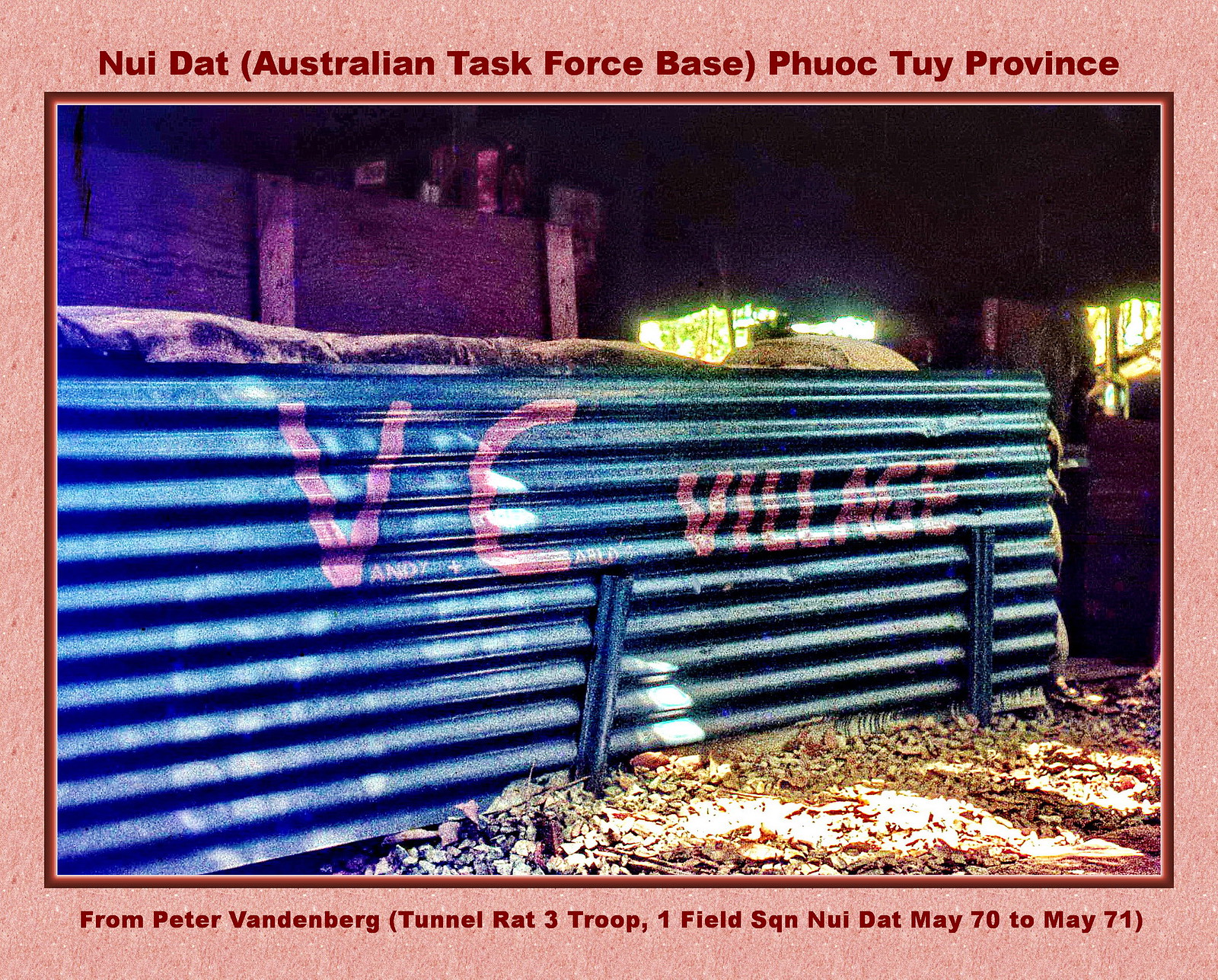The image depicts a hand-constructed fort-like structure set during the Vietnam War, positioned directly in the center of a color photograph that is in landscape orientation. The photograph is framed by an off-pink border with dark red text at the top and bottom. The headline at the top reads "Nui Dat (Australian Task Force Base) Fuak Tui Province," and the caption at the bottom reads "From Peter Vandenberg (Tunnel Rat 3 Troop, 1 Field SQN, Nui Dat, May 70 to May 71)." 

In the foreground, there is a distinctive corrugated metal wall painted blue, displaying the words "VC Village" in pink paint. This wall, reinforced by several vertical and horizontal supports, runs diagonally from the lower left to the upper right. Behind the metal wall, a wooden structure with vertical slats and windows is visible, adding to the scene's complexity. The setting appears to be an outdoor area at night, evoking the tension of a wartime environment. The photograph’s detailed color palette includes shades of pink, maroon, brown, purple, blue, red, yellow, light brown, and a hint of green, enhancing the realistic and immersive depiction of the scene.